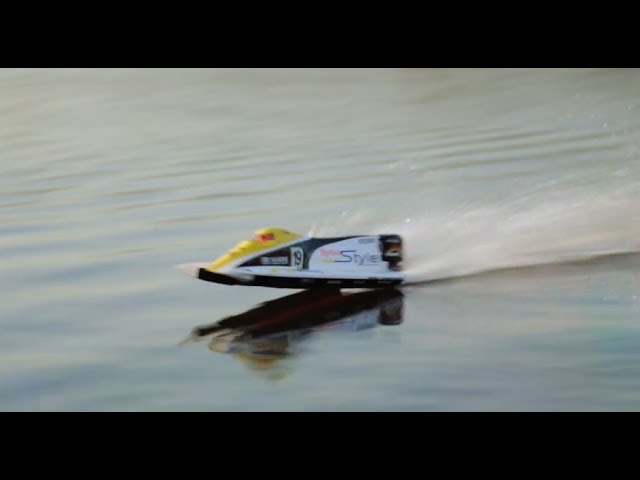The image captures a dynamic scene of a toy-like watercraft, likely controlled by remote control, skimming across a body of water. The vessel, which appears small due to the absence of surrounding objects for size comparison, is slightly blurred, adding to the sense of motion. It sports vibrant colors, with the top section being yellow with a hint of red, and the rest adorned with black and white markings. There is text on the toy that reads "Style" alongside the number "19." As it speeds across the water, it creates a noticeable wake and spray, demonstrating its swift movement. The craft is partially lifted above the water's surface, almost as if it is attempting to take off. Its dark shadow is visible on the water below, further emphasizing its elevated position.